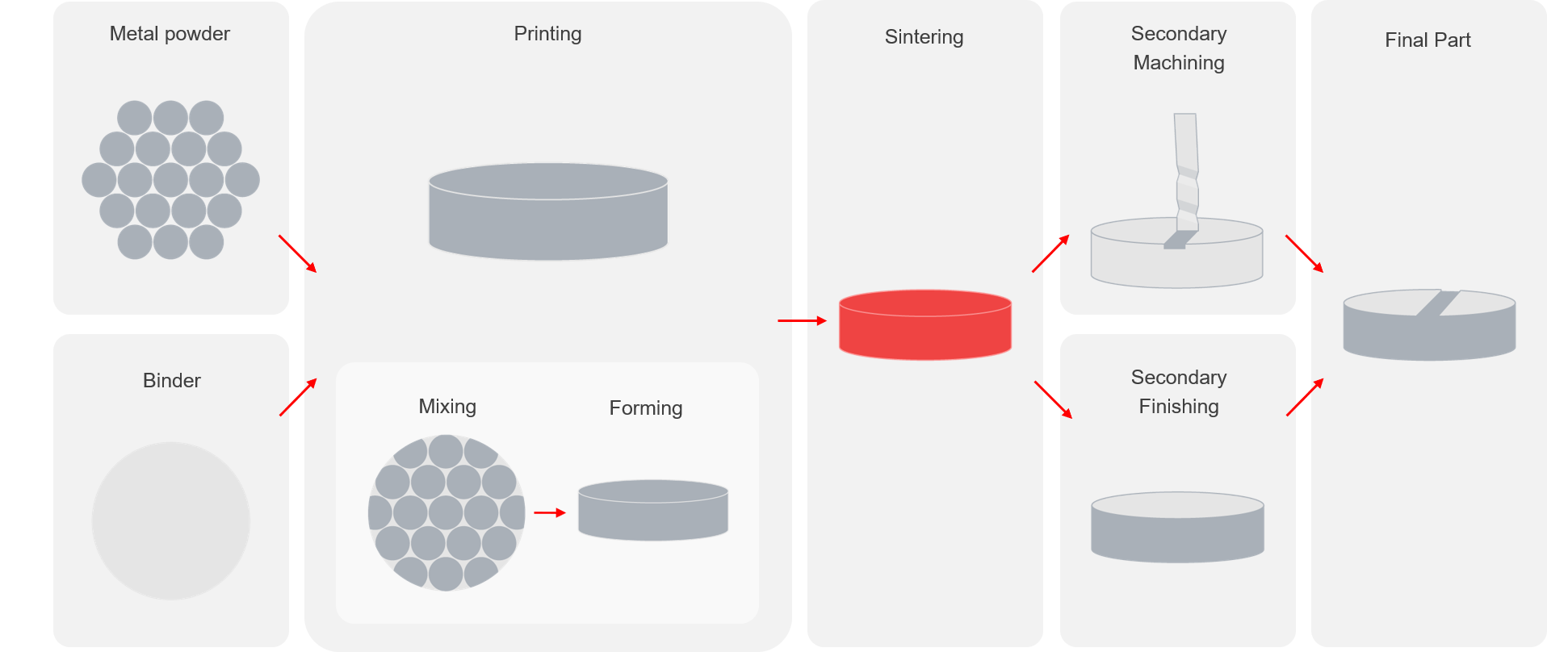This digital image is a detailed scientific chart with rounded rectangles organized to describe a metal component manufacturing process from left to right. The chart is divided into seven sections of varying rectangular sizes with illustrations and black text. 

Starting on the top left, a small rectangle labeled "metal powder" features an image of metal powder alongside circles, and a red arrow pointing to a large rectangle to its right. Beneath it, another small rectangle labeled "binder" contains a gray circle and similarly points to the large rectangle. The large rectangle, titled "printing," depicts the metal powder mixing with the binder and highlights the steps of "mixing" and "forming" through images and text. 

To the right of the large rectangle is a tall, thin rectangle labeled "sintering," showcasing a red cylindrical or disc-shaped object at the top. Further right, two small stacked rectangles are labeled "secondary machining" and "secondary finishing" respectively, each within an illustration of machinery steps. The final tall, thin rectangle on the far right is labeled "final part" and illustrates the completed metal part.

Color usage in the chart is primarily gray, with notable uses of red and white to highlight specific processes and transitions, illustrating the journey from raw material to finished product.